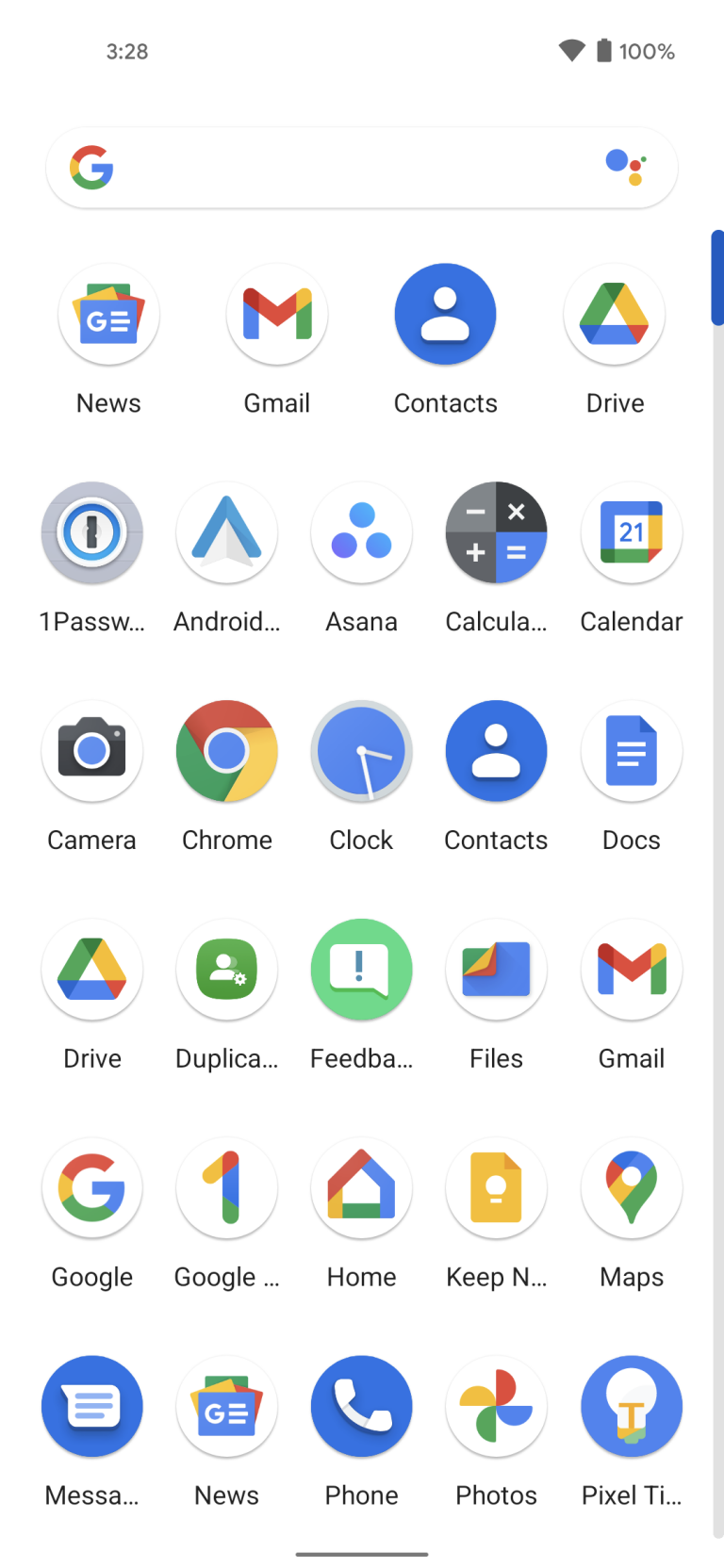The image is a screenshot of a mobile phone display showcasing a list of installed applications. The background is predominantly white. Positioned at the top-left corner, the time is shown as 3:28 in black text. On the upper right, there are icons for reception/Wi-Fi, battery status indicated as 100%, and the battery icon itself.

Directly below these indicators, there is a search bar featuring the Google 'G' logo on the left. On the right side of the search bar, there are three colored dots: blue, red, and yellow, likely representing Google Assistant or microphone input. There is also a progress bar running along the right side of the screen.

In the main section of the display, the applications are arranged in a grid format. The grid consists of four columns across and six rows down, featuring a variety of app icons. These include:

- News
- Gmail
- Contacts
- Drive
- Calculator
- Calendar
- Camera
- Chrome
- Clock
- Docs
- Files
- Home
- Maps
- Messaging
- Phone
- Photos